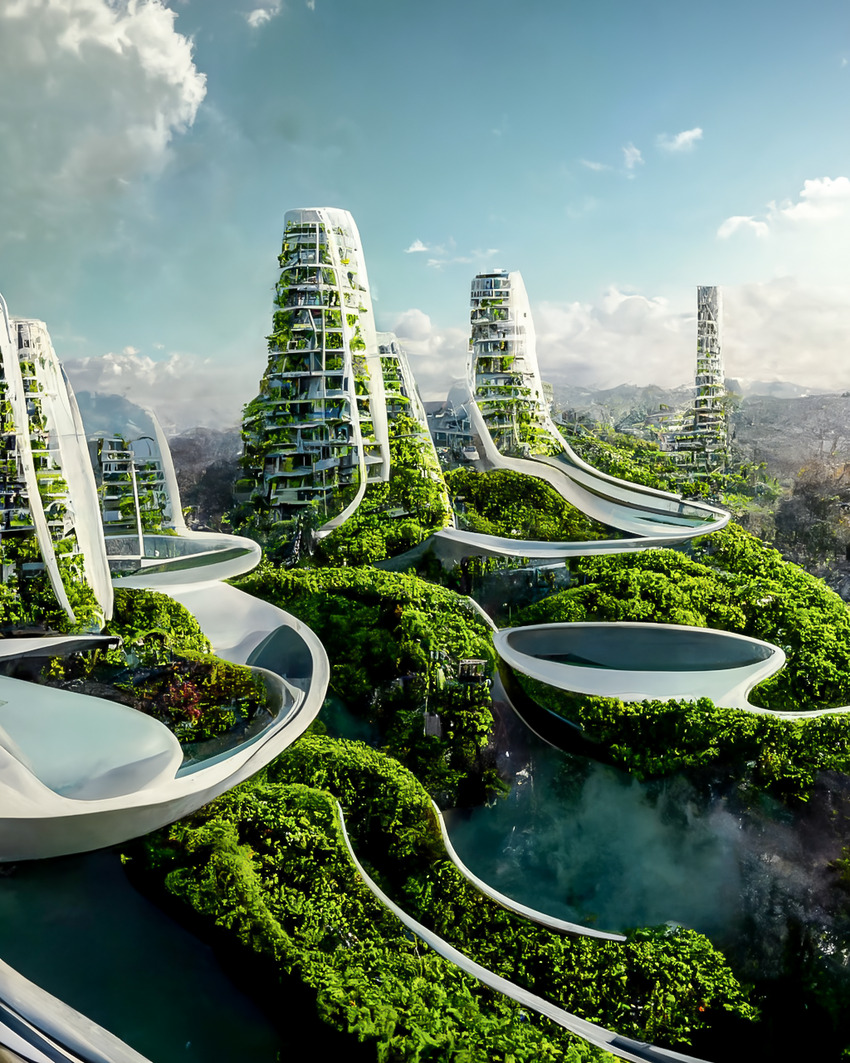The image showcases a futuristic city seamlessly integrated into the countryside, set against a backdrop of a blue sky adorned with gray clouds. Dominating the foreground are several sleek white towers, approximately 20 stories high, that epitomize advanced architectural design. These towers are adorned with abundant vegetation and plant life, suggesting an eco-friendly approach to urban living. To the left, two barely visible buildings rest on a silver platform, which also hosts some greenery. Adjacent to these, a prominent tower stretches upwards, leading to a meandering road that curves around to connect with another distant structure. This far-off building appears taller and more imposing, albeit shrouded in a misty aura.

The lush vegetation continues at ground level, where a silver circular road encircles a black dot, creating a focal point in the composition. The image also hints at a floating effect, as though the entire scene is suspended in mid-air. The presence of moisture and potential mountain silhouettes in the background enhance the ethereal quality of the setting. The blue-turquoise hues at the base of the structures may suggest water, adding to the utopian ambiance.

This artist’s or AI-generated rendition envisions a harmonious blend of nature and futuristic architecture. It illustrates the transformative effects of integrating plant life into urban designs, contributing to a greener, less polluted environment. Overall, the depiction not only emphasizes the aesthetic beauty but also conveys a hopeful vision of what future cities could achieve by prioritizing environmental sustainability.